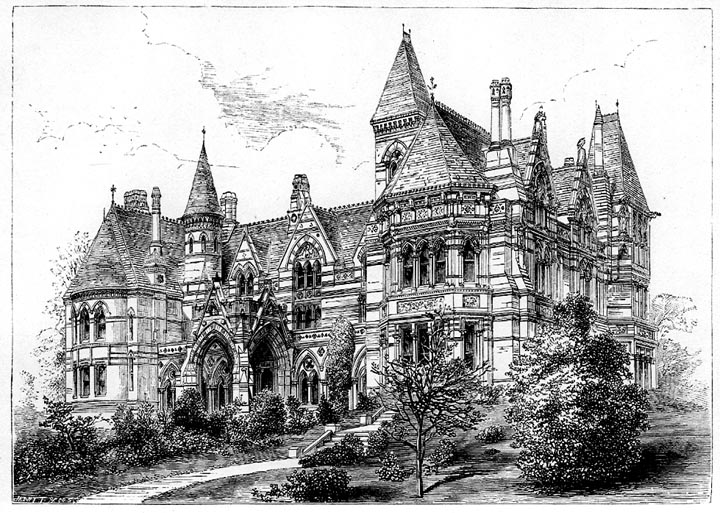This is an intriguing black and white illustration, likely drawn in pencil, that meticulously depicts a grand, old-fashioned building with elements suggesting it could be a Victorian or Gothic-style house, or even a castle. The structure is notable for its intricate and elaborate design, featuring multiple roof lines, peaks, and tall, pointy towers with distinctive round sections integrating tall windows. The image is wider than it is tall and framed by a penciled-in black border. The foreground highlights a meticulously landscaped area with a walkway lined with bushes and a few trees, some appearing bare as if in winter, adding to the drawing's intricate detail. The sky above is mostly white, with only the faint outlines of clouds, enhancing the timeless and serene quality of the scene. This intricate and beautifully rendered illustration could easily grace the front of a postcard or serve as a vintage keepsake from a bygone era.